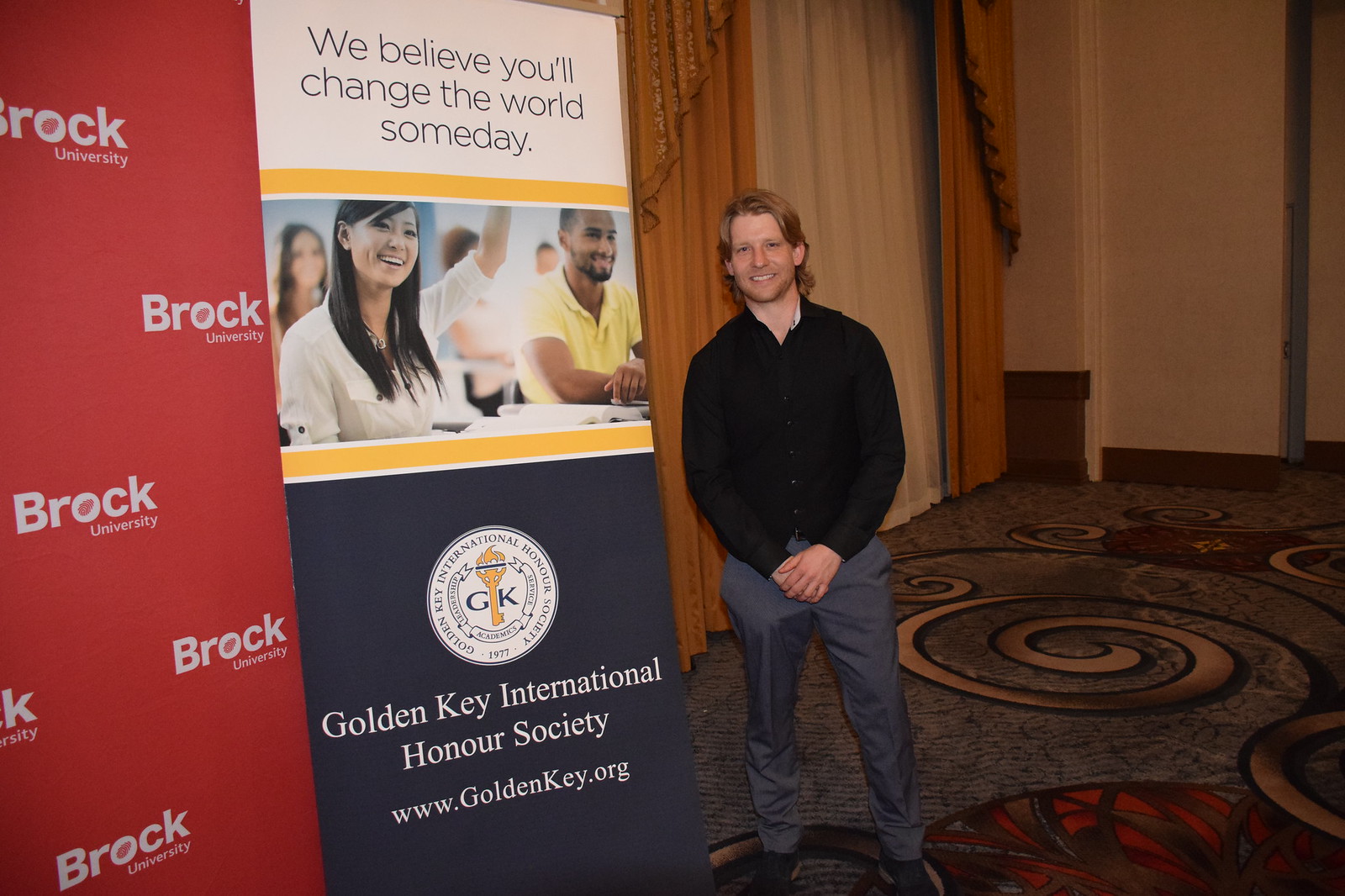A young man stands at the center of the image, clad in black shoes, gray dress pants, and a black button-up shirt with a collar and long sleeves. His dirty blonde hair falls to around his neck and shoulders. He stands on a carpet with various tan-colored swirls bordered with black lines. Behind him is a gold and yellow curtain wall. To his left is a tall banner that is blue, white, and yellow. The top part of the banner features text in black font on a white background that reads, "We believe you'll change the world someday." Below this text is a picture of a classroom filled with adults, one person raising their hand. The bottom section of the banner is dark blue with white font and shows the logo of the Golden Key International Honor Society, along with the text "Golden Key International Honor Society" and "www.GoldenKey.org." The far wall on the right side of the image is visible, painted white with brown trim. On the left, partially visible, is a step-and-repeat backdrop that is black with white text reading "Brock University."